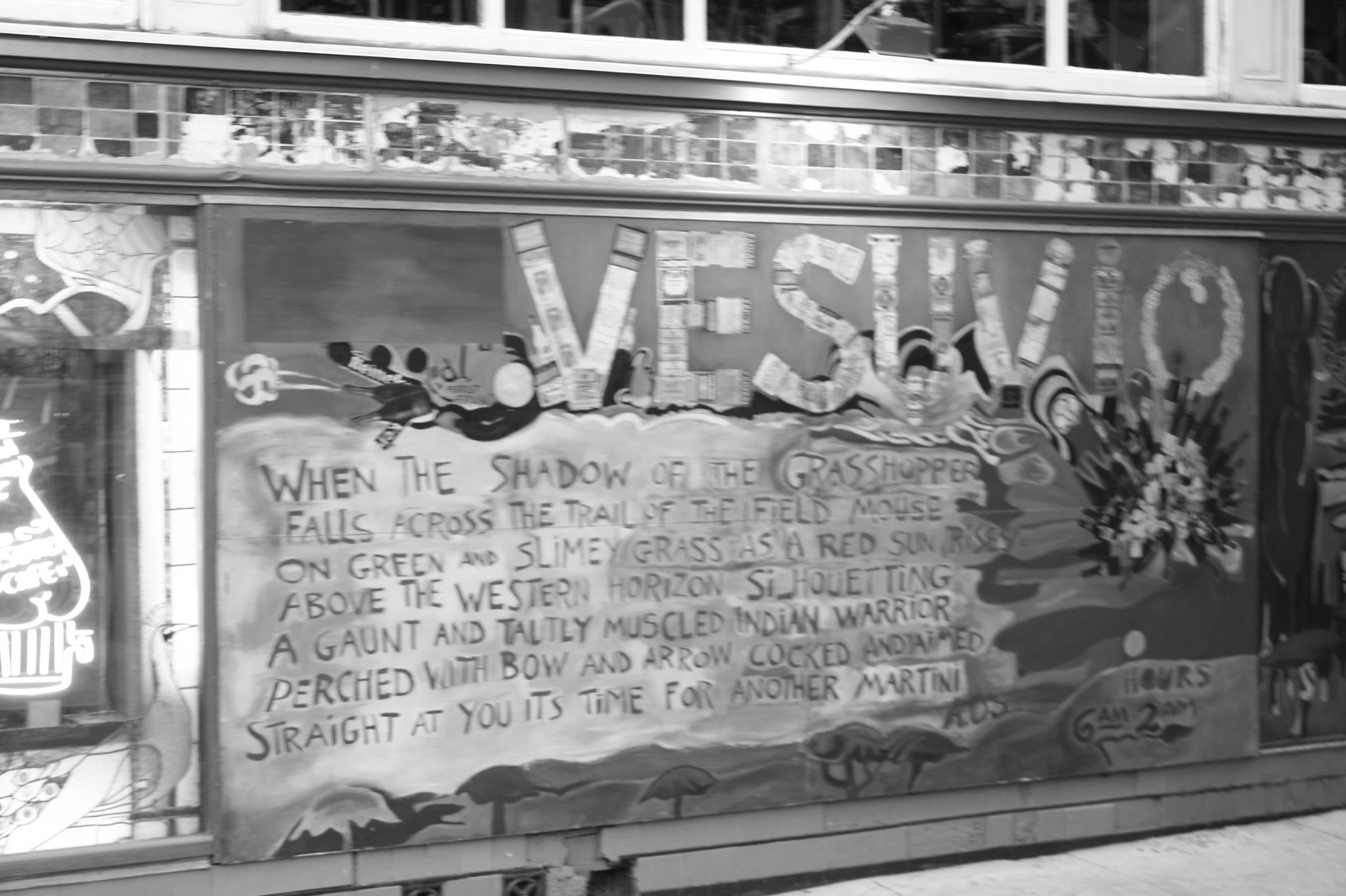This detailed black and white photograph captures an outdoor mural located on a city street. The mural, positioned prominently in the center of the image and spanning from left to right, appears on a tile wall beneath some sharp windows. Above the artwork, a light fixture illuminates the mural, lending it an eclectic and mysterious ambiance. The mural features the text "Vesuvio" at the top, with an intricate and poetic passage below that reads: "When the shadow of the grasshopper falls across the trail of the field mouse on green and slimy grass, and a red sun rises above the western horizon, silhouetting a gaunt and tautly muscled Indian warrior perched with bow and arrow cocked and adorned straight at you, it's time for another martini." This elaborate mural also includes drawings of trees at the bottom, indicating it serves as a sign for a business named Vesuvio.